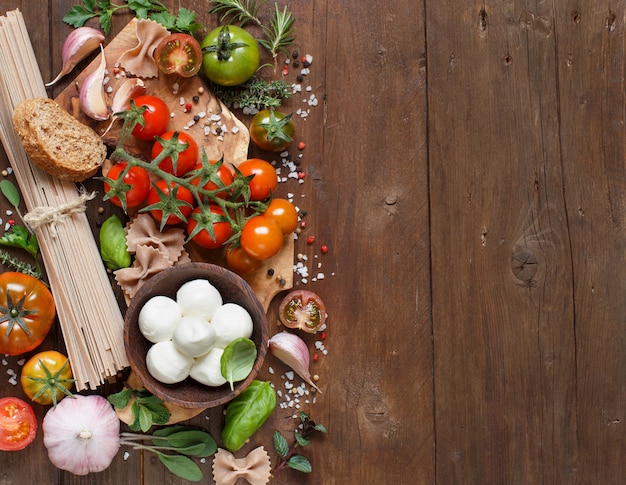This overhead shot captures a dark wooden table with noticeable vertical lines resembling floorboards. The image is split into two distinct sections: the right half showcases the rich, bare wooden surface, while the left half is densely packed with an array of fresh ingredients. Among the vibrant collection, we see a variety of tomatoes—including cherry tomatoes on the vine, green tomatoes, and sliced tomatoes—surrounded by bulbs of garlic and shallots. A rustic bundle of linguine pasta tied with a piece of rope, alongside a wooden bowl brimming with mozzarella cheese balls, adds to the culinary assortment. Scattered around are sprigs of fresh herbs such as rosemary and thyme, along with grains of salt and pepper. Notably, there's also a slice of wheat bread and various pasta shapes like butterfly noodles. This composition suggests the initial preparations for a hearty homemade pasta dish, set against the warm, earthy tones of the wooden table.